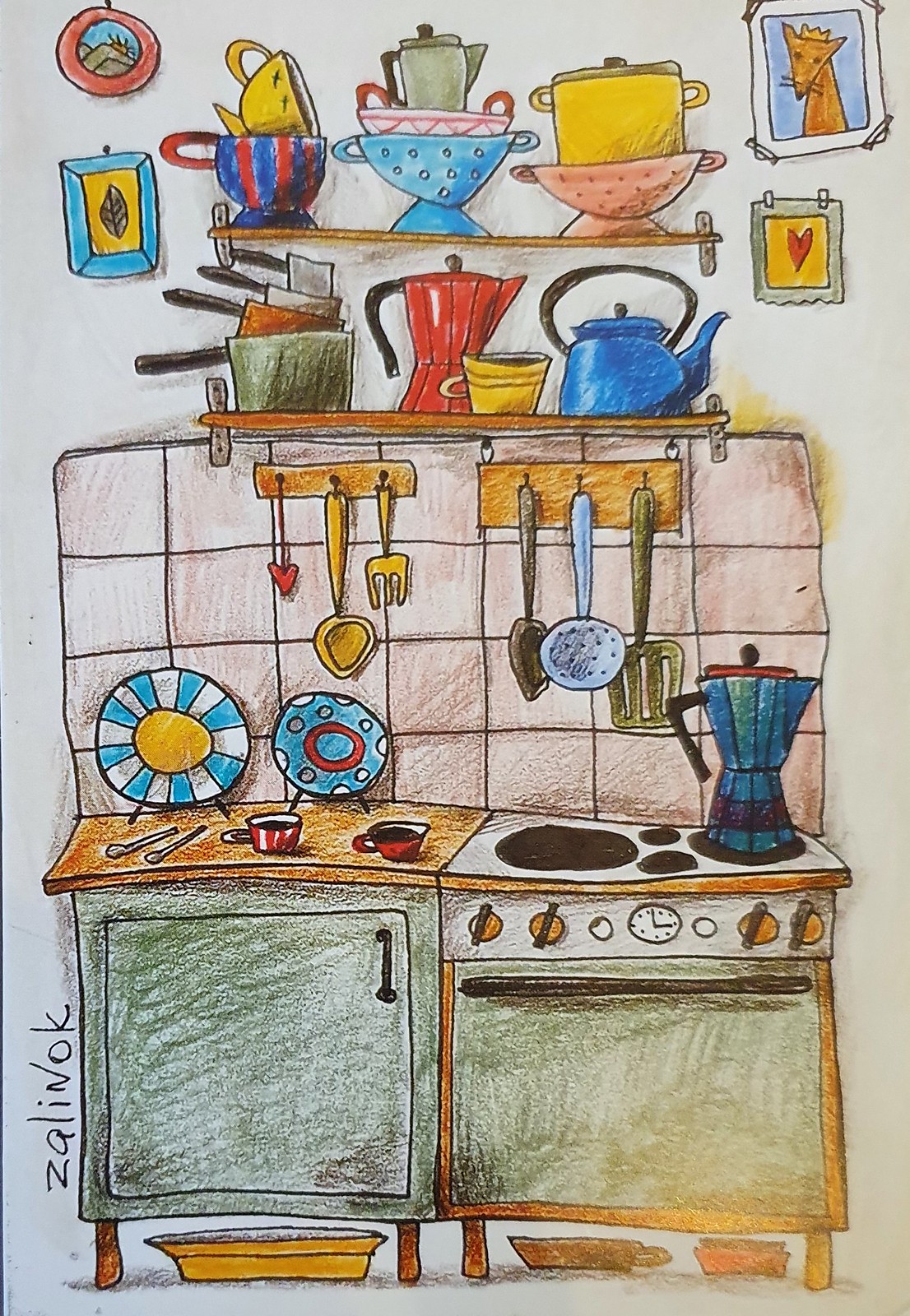This is a detailed, vibrant sketch by the artist Zalanok, prominently signed in the corner. The drawing, executed with pen and enhanced with colored pencil or crayon, depicts an intricately cluttered kitchen scene full of character and color. Central to the scene is an uneven kitchen countertop, surfaced partially with wood. To the right, a stove with black burners and a blue pot with a black handle sits atop it. Adjacent is a green cabinet with a black handle, possibly a refrigerator, topped with a wooden counter.

The kitchen is replete with details: decorative plates adorn the walls, including one with a yellow ball and blue rays and another blue plate with yellow and white polka dots, encircled by red. Red mugs filled with black liquid, various spoons, and other kitchen essentials are strewn across the wooden countertop. Above the countertop, a wooden rack holds an assortment of hanging utensils, such as a green spatula, various spoons, and a fork, while shelves above are precariously stacked with pots, pans, teapots, and colanders in various colors.

Adding to the ambiance, the walls are adorned with framed pictures, including a whimsical portrait of a dog wearing a crown and another with green leaves. This kitchen comes alive with its detailed and expressive crayon strokes, making it a rich tapestry of domestic life.